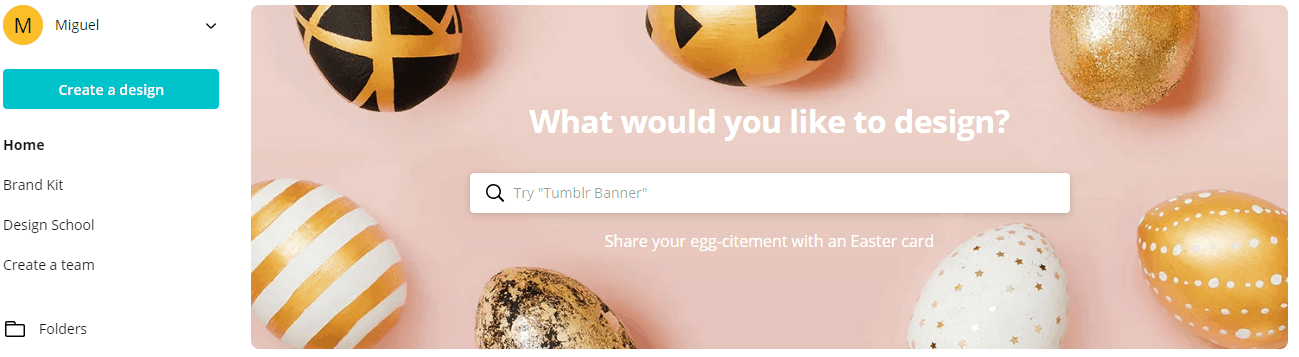The screenshot captures a midsection of a website, where the header is not visible, leaving the specific site unidentified. Dominating the layout is a photograph taking up about three-quarters of the image. The photo is a horizontally elongated rectangle set against a background that transitions between a light lavender and pink hue. The central visual elements are ornate Easter eggs. At the top of the photo, partially visible, are three elaborately decorated eggs. The one on the left is gold and black, the central egg is gold with black triangles, and the rightmost egg is a solid gold color.

The bottom part of the photo features more decorative Easter eggs. In the lower left corner, there is a gold and white striped egg, followed by a gold and black egg with a stonelike appearance. Next to these, there is an egg with tiny gold dots on a white background, and in the lower right corner, a solid gold egg with white dots catches the eye.

Above the photo, in white text, is a headline that reads, "What would you like to design?" Below this headline is a search box, a long white rectangle, with a magnifying glass icon on the left side and the prompt “Try Tumblr banner” inside the box. Beneath the search box, another text line reads, "Share your egg excitement with an Easter card."

On the left side of the screenshot, there is a white sidebar. At the top left corner of this sidebar, it says "Miguel" next to a gold circle with a black letter "M." Below this, a blue rectangle with white text prompts "Create design." Further down the sidebar, against the white background, more menu items are listed: "Home," "Brand Kit," "Design School," "Create a Team," and at the very bottom, "Folders."